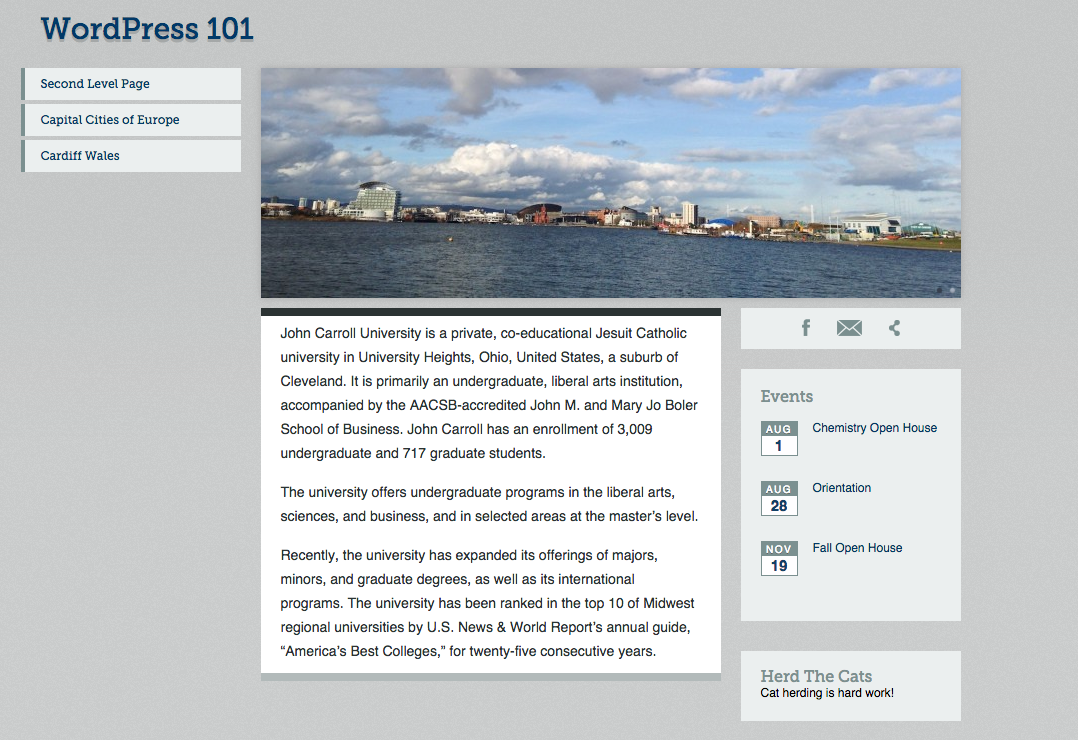This screenshot features a WordPress page with a gray background. At the top left, "WordPress 101" is prominently displayed in large, dark blue font. Directly below this title, there are three categories listed vertically within gray boxes that are accentuated with blue lines on their sides. These categories are labeled in the following order: "Second Level Page," "Capital Cities of Europe," and "Cardiff, Wales."

To the right of these categories, a large rectangular image captures a picturesque seaside city. Beneath this photo, on the bottom left, sits a sizable white box containing information about John Carroll University.

Just below the image's bottom right corner, a smaller rectangular box contains icons for Facebook, mail (an envelope icon), and sharing options. Following this, another large white box labeled "Events" in the top left corner displays three calendar entries. These entries are listed in chronological order: "August 1st, Chemistry Open House," "August 28th, Orientation," and "November 19th, Fall Open House," with the dates on the left and the event titles to their respective right.